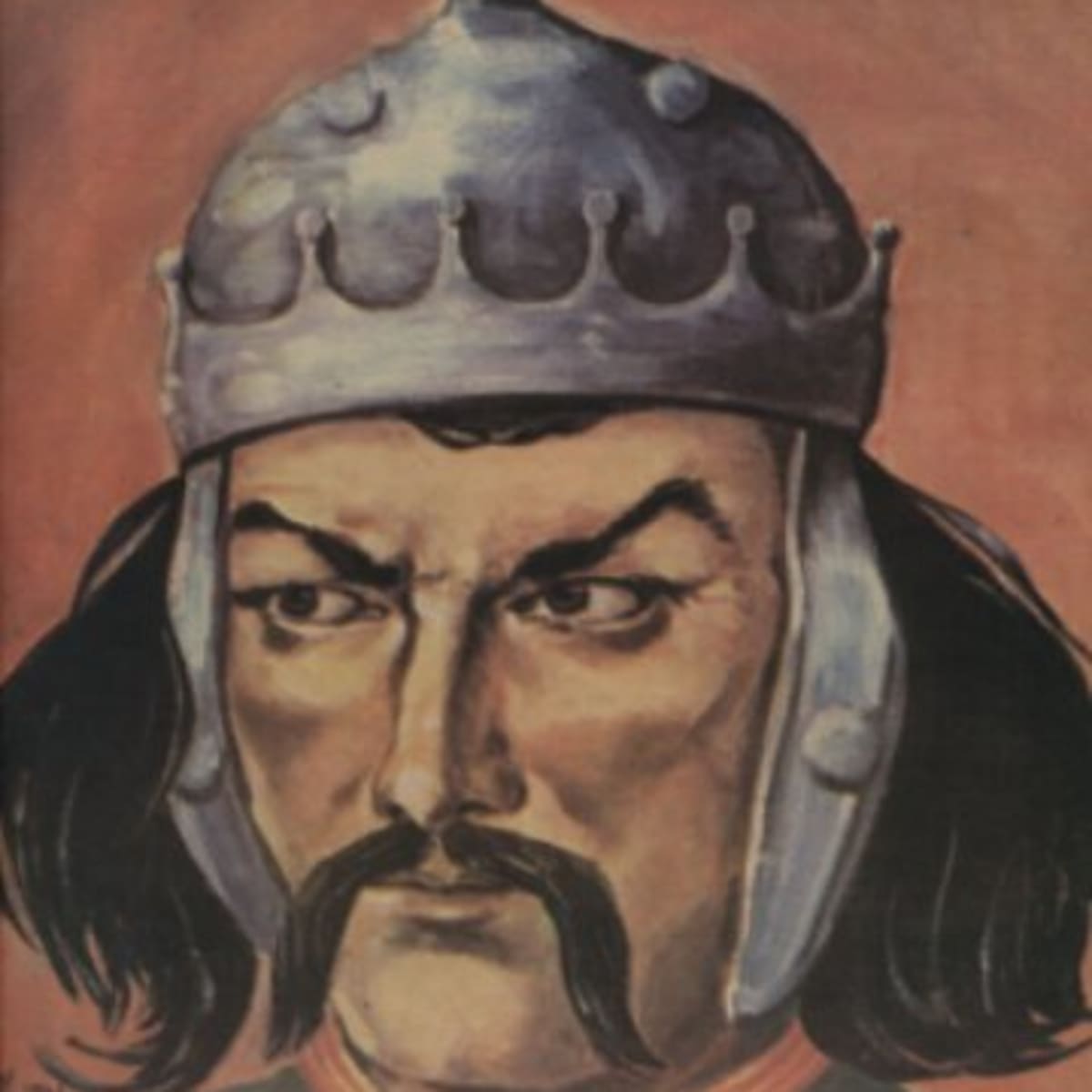This is a highly detailed close-up illustration of a man’s face, capturing the essence of an Asian warrior. His skin tone is predominantly white with a slight darkness around the cheeks and sides of the chin, emphasizing his strong facial structure. He has a long, pronounced nose and high, defined cheekbones. His arched, sloping eyebrows give him a somewhat menacing expression. He sports a distinctive black Fu Manchu mustache that extends below his chin.

The man’s head is adorned with a silver helmet that resembles a crown, featuring a domed top and metal pieces descending to cover his ears. His long black hair flows down to his shoulders, framing his face. The background of the image is washed out with a reddish-pink hue, enhancing the dramatic tone of the illustration.